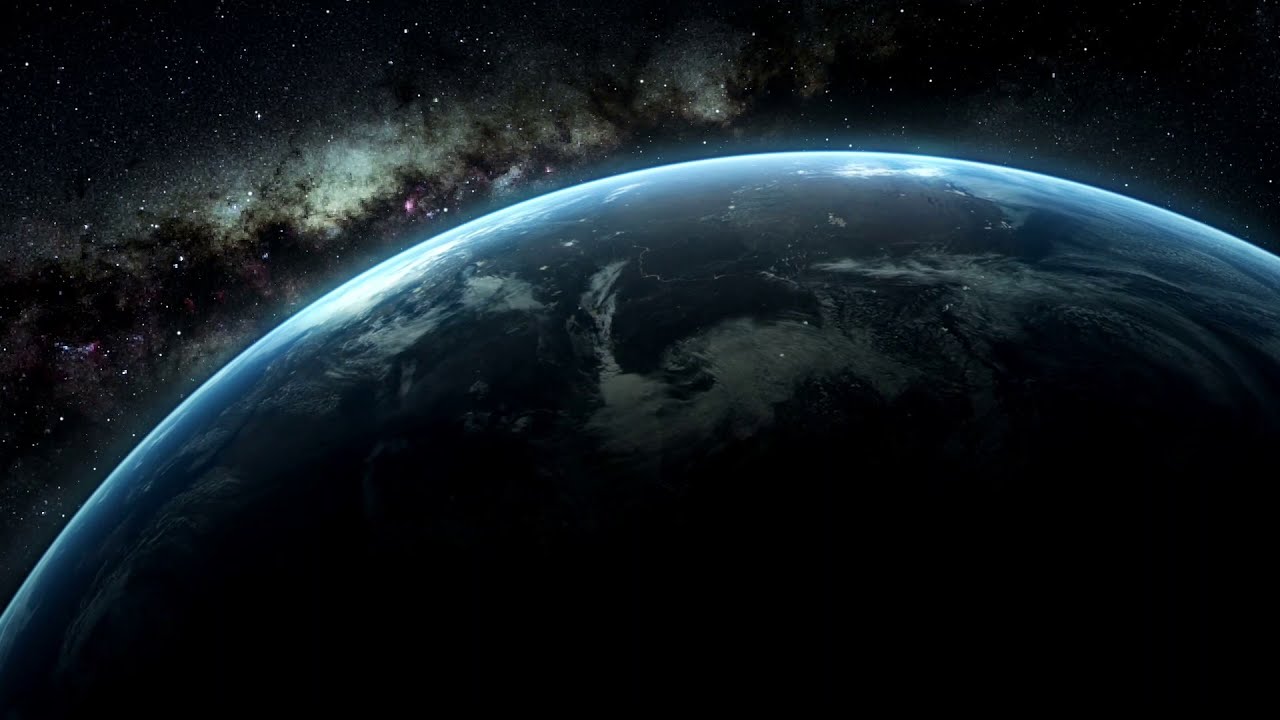The image captures a stunning view of Earth from outer space, where the planet is displayed partially, with a vibrant blue outer edge. The illuminated arc of Earth rises from the lower left to just above the halfway point on the right side, revealing detailed land and water formations along with spirals of clouds. The overall scene is dark, evoking a sense of nighttime, and is set against a backdrop of the Universe. The dark sky is filled with bright stars, patches of clouds, and scattered pink and white dots representing constellations. The vivid colors in the image range from deep black to white, blue, and green, with hints of pink, providing a clear and mesmerizing visual experience.